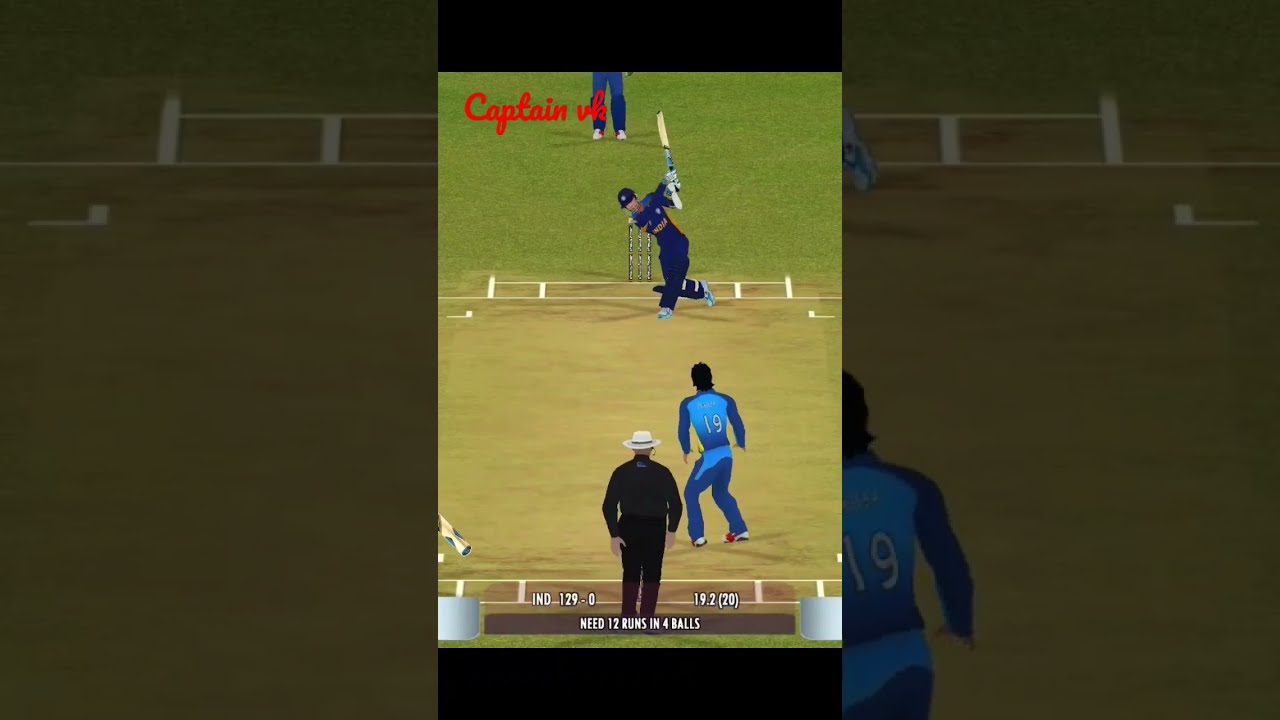The image captures an intense moment in a cricket video game, featuring two main players on the field. In the foreground, a player in an all-navy blue uniform with golden yellow lettering is mid-swing, holding a bat, indicating he is the batsman. Nearby are stumps, indicating the wicket he is protecting. Across from him stands the bowler, dressed in a sky-blue jersey with navy blue sleeves and pants, identifiable by the number 19 on his back. Behind the bowler, a referee clad in a black long-sleeve shirt, black pants, and a beige hat observes the game. The pitch is framed by a green grassy field and white painted lines marking the cricket crease. The phrases "Captain VK" appear in a large cursive red font in the top left corner of the image. Additionally, there are statistics displayed at the bottom of the image reading "129-0," "19.2," "20" in brackets, and "12 runs needed in 4 balls," indicating the game’s current scenario. The detailed depiction is also inset within a transparent gray overlay, adding emphasis and focus to this critical moment in the match.